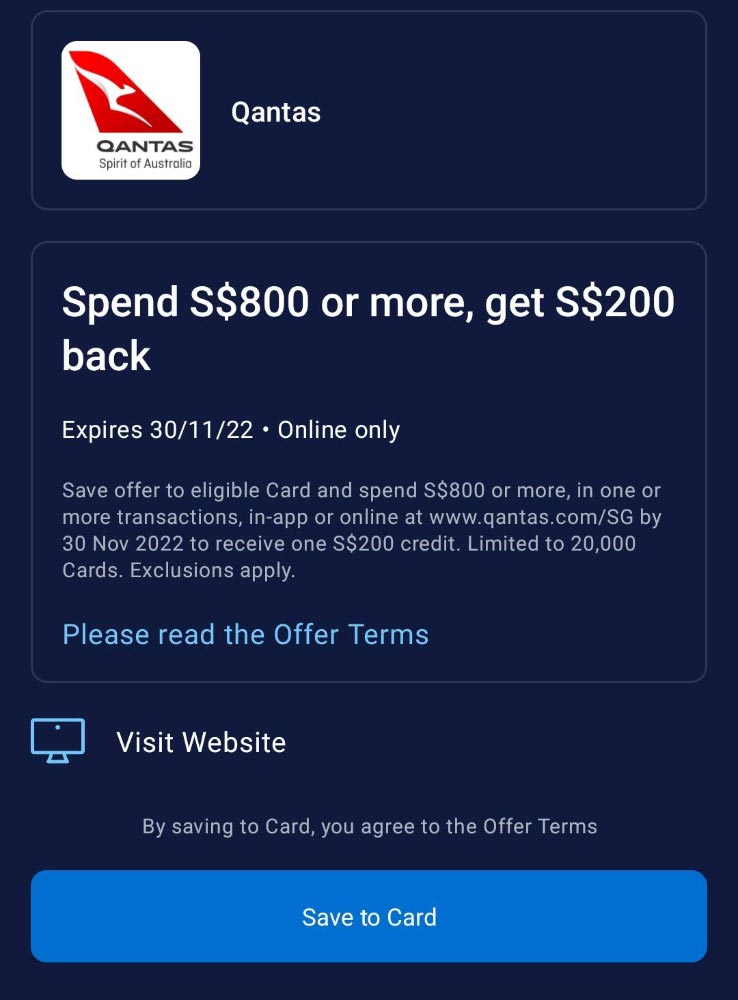The image is an advertisement for a promotion by Qantas Airlines. Against a dark blue background, two text boxes are prominently displayed. The first text box contains the Qantas logo, which features a red airplane tail and a white kangaroo, accompanied by the tagline "The Spirit of Australia." 

Below the logo, the second text box provides details of the offer: "Spend 800 SGD or more and get 200 SGD back," with the expiration date listed as November 30, 2022. The offer is applicable exclusively for online purchases made at www.qantas.com/sg by November 30, 2022. To avail the offer, customers must save it to an eligible card and spend 800 SGD or more in one or multiple transactions. The promotion is limited to the first 20,000 cards and certain exclusions apply, so customers are encouraged to read the full offer terms. 

Beneath this text, there is an image of a computer with a prompt to "Visit Website," followed by an advisory that saving the offer to the card implies agreement to the offer terms. A large blue button labeled "Save to Card" is positioned at the bottom, inviting action from the viewer.